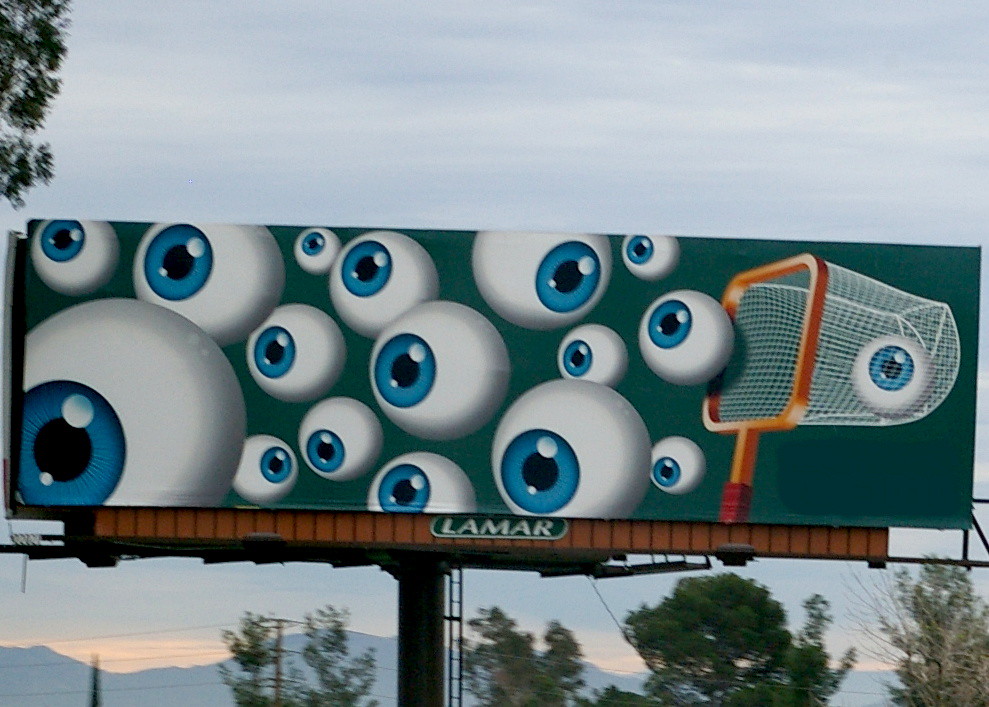The image features a billboard with a surrealistic artwork depicting a net capturing large eyeballs. The eyeballs are highly detailed, characterized by their white spheres, vivid blue irises, and reflective white spots on their surfaces. The net, positioned on the right-hand side, has a white weaved basket with an orange frame and handle, seemingly tipped to the right by the weight of a captured eyeball. The billboard has a dark green or blue background, with the world "Lamar" inscribed below, indicating the company that owns it. The setting includes a ladder leading up to the billboard's pole, with the surrounding environment showcasing a sunset sky, telephone poles with wires, and green-topped trees. Mountains loom in the distant background, adding further depth to the evening scene.